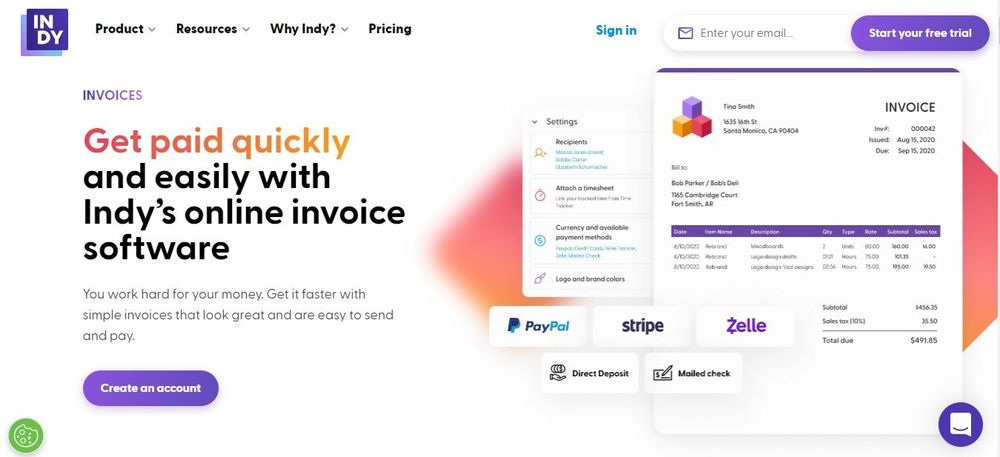The image showcases an Indie website interface, characterized by a vibrant and inviting aesthetic. The site features a predominantly white background accentuated with splashes of purple and pink hues, reflecting its creative invoice software branding.

On the left side of the image, the Indie logo stands out, presented in bold white capital letters against a raw blue background and enclosed within a small square. Adjacent to the logo, the top navigation menu includes options such as "Product," "Resources," "Why Indie," and "Pricing."

Further to the right, users can access the sign-in option, featuring an email input box alongside a call-to-action button labeled "Start your free trial." 

Returning to the left, the next section prominently displays the word "INVOICES" in all caps. Directly beneath, a caption reads: "Complete quickly and easily with Indie's online invoice software. You work hard for your money; get fast and simple invoices that are great, and are easy to send and pay."

Moving right, there is a segment of informational boxes. One smaller box offers setup options for viewing preferences on the site, while the larger box prominently features a sample invoice. This mock invoice includes critical details such as the sender's name and address, the issuing date, the recipient's name ("Bill To"), and additional invoice particulars.

The sample invoice also contains clickable links to payment platforms like PayPal, Stripe, and Zelle, along with billing options such as direct deposit and mailed checks.

At the bottom of the image, options are available to create an account or send a message, indicated by a small message icon.